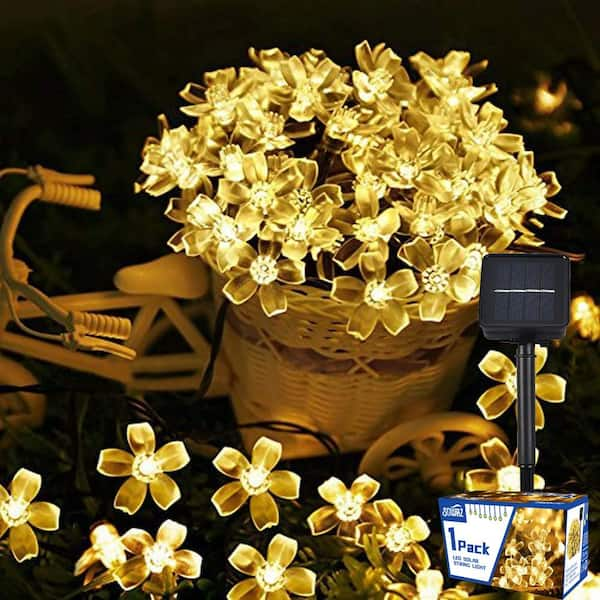The image depicts a bicycle in the background with a white wicker basket affixed behind its seat, filled with lit, golden-yellow flower-shaped lights. The background is entirely black, making the illuminated flowers stand out vividly. These flowers have lights in their centers and appear delicate and elegant. On the right side of the image is a stand featuring a white box with blue trimming on the sides, displaying the text "one pack" in blue letters along with a close-up picture of the flower lights. A black cord can be seen running near the basket, suggesting the lights might be solar-powered. The overall scene exudes a sense of dainty sophistication, likely aimed at showcasing a product that blends aesthetics with sustainable lighting.